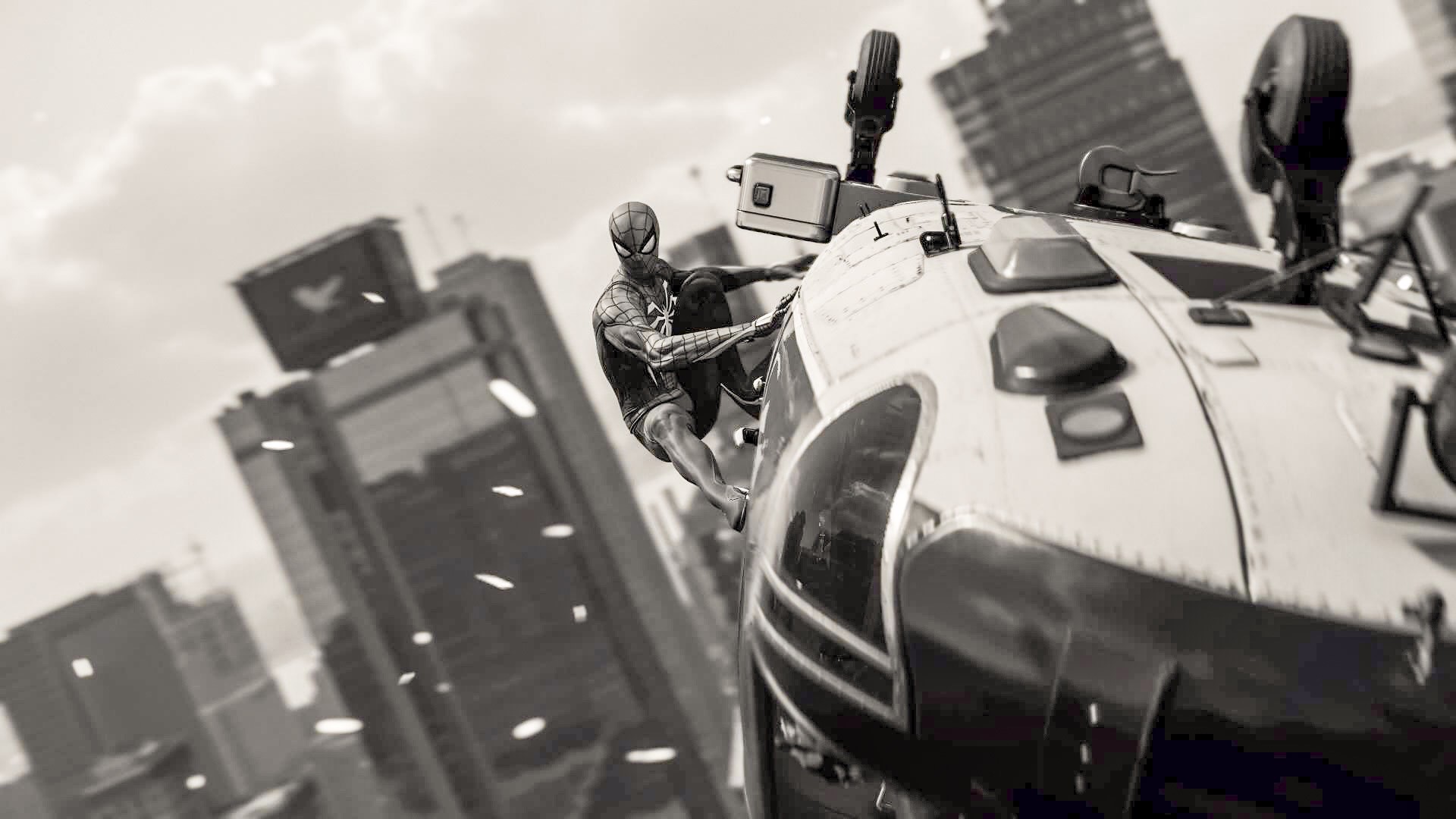In this black and white computer-generated image, Spider-Man is seen clinging determinedly to the side of an upside-down helicopter, which has its wheels visible on top. The helicopter has a white underbelly and a dark nose, contrasting against a cloudy, stormy New York City backdrop. Skyscrapers fill the background, some angled due to the perspective. A prominent building features a large black container with a bird logo, reminiscent of the Twitter logo. Floating white objects stream down to the left, adding to the chaotic atmosphere of the scene. The image appears to be from a Spider-Man game or movie, capturing an intense moment where Spider-Man is trying to save people in the helicopter.